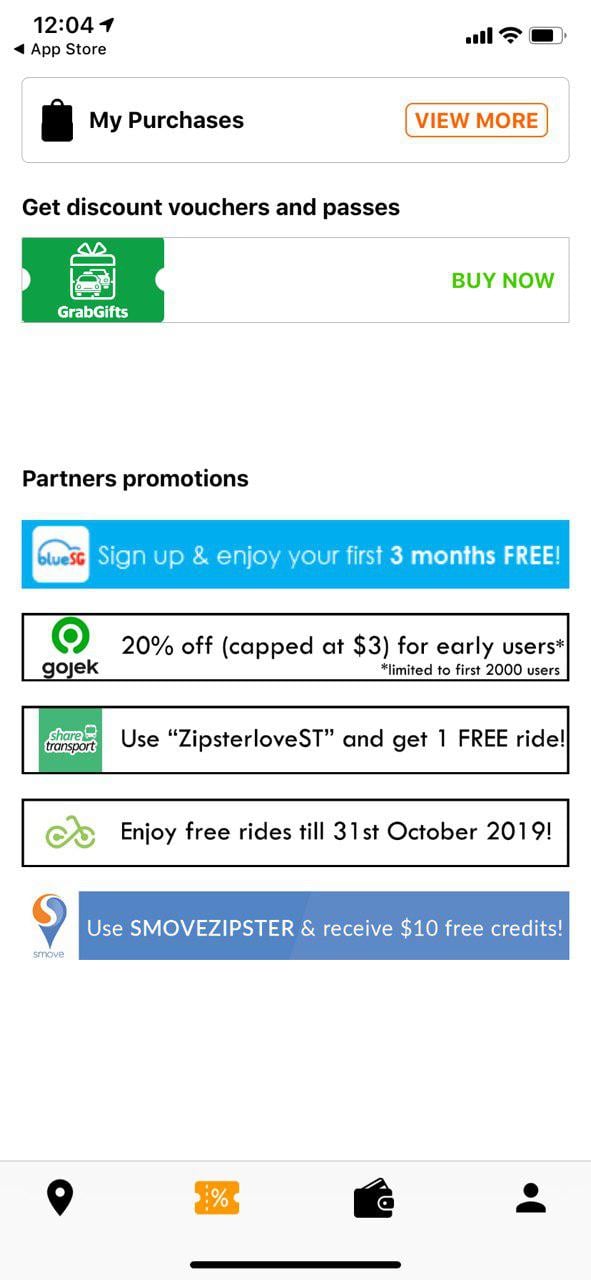The image is a screen capture of a smartphone's display. In the top-left corner, the time reads 12:04, and the device is connected to the App Store with four bars of signal strength and approximately 75% battery life. At the top of the screen, there is a navigation bar with a shopping bag icon labeled "My Purchases" on the left, and a button on the right with orange text stating "View More."

Below the navigation bar, there's a black text header offering discount vouchers and passes accompanied by a coupon icon. The text "Buy Now" is displayed prominently.

Further down, the screen displays a section titled "Partner Promotions" in black lettering. This section contains a list of promotions:
1. A blue banner featuring a logo that appears to be "SC" or "SG," with the text "Sign up and enjoy your first three months free" in white lettering.
2. A rectangular promotion offering "Gojek 20% off capped at three dollars for early users, limited to the first 2,000 users."
3. A promotion featuring a green logo stating "Use Zipter Love ST and get one free ride."
4. An offer with a green bike icon that reads "Enjoy free rides until 31st October 2019."
5. Another promotion, "Use S Move Zipster and receive $10 in free credit."

The screen suggests that the user is exploring various ways to save money through different promotional offers.